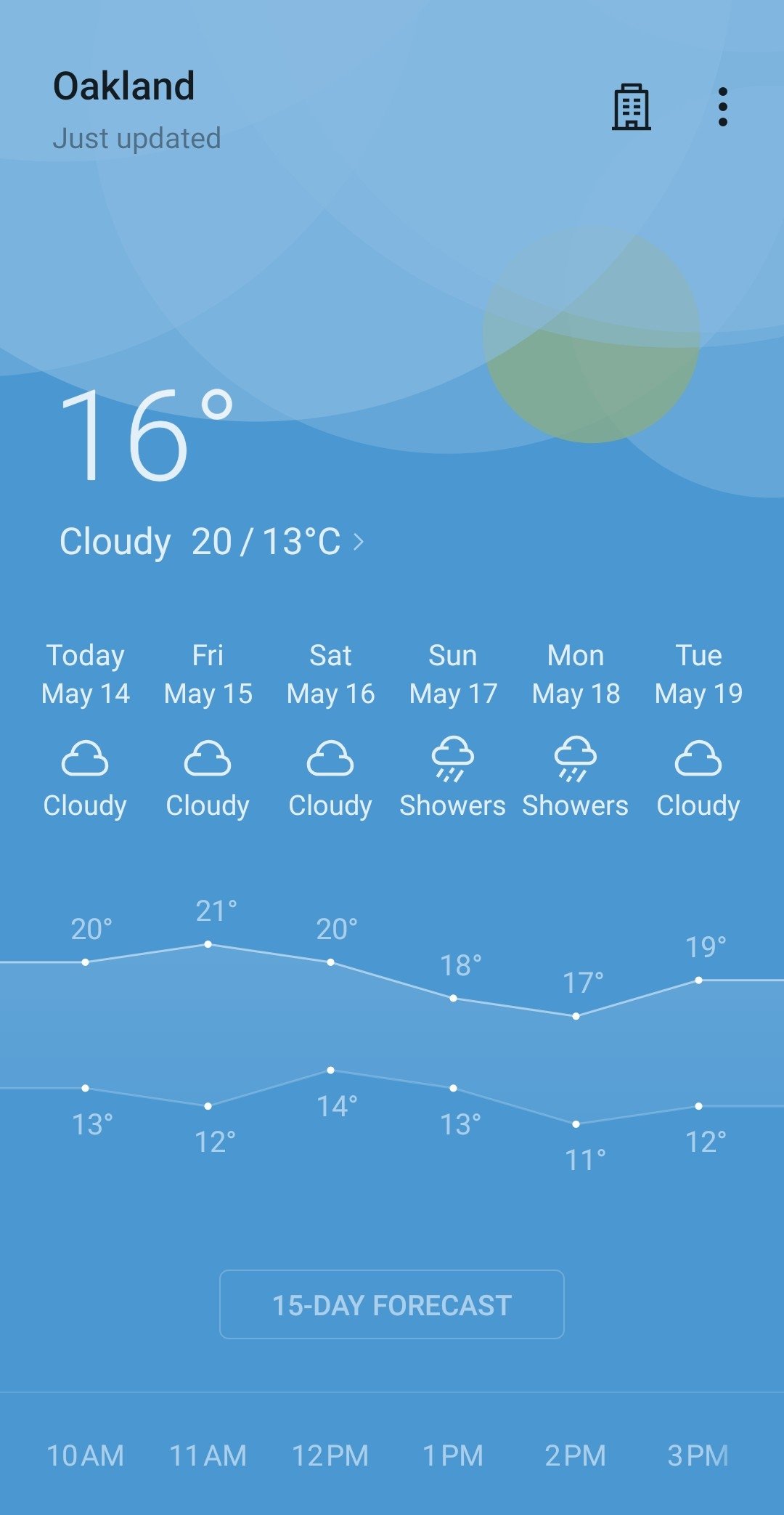This screenshot showcases a weather forecast for Oakland. The background features a light blue sky transitioning into lighter blue cloud-like patterns at the top, with a small yellow circle on the right side representing the sun partially hidden behind the clouds. 

In the upper left corner, the word "Oakland" is displayed in black text, with "just updated" shown below it. The upper right corner includes an icon resembling a skyscraper, accompanied by three vertical black dots aligned to its right.

Centrally positioned, the temperature is prominently displayed in white text as "16°C," directly below which it indicates "Cloudy," with a range of "20/13°C." An arrow directed to the right follows this information.

The daily forecast is listed beneath, starting with "Today, May 14th," labeled as "Cloudy" with a small cloud icon. This pattern continues with "Friday, May 15th," "Saturday, May 16th" all labeled "Cloudy" with corresponding icons. "Sunday, May 17th" and "Monday, May 18th" show a cloud with rain for "Showers.” Ending with "Tuesday, May 19th," again labeled "Cloudy."

Further down, there is a temperature graph depicting fluctuations over the upcoming days: temperatures range from 20 to 21, then back down to 20, 18, 17, and 19 degrees Celsius. The corresponding low temperatures track from 13 to 12, up to 14, back to 13, 11, and 12°C.

At the center near the bottom, a rectangular button labeled "15-day forecast" is displayed, followed by hourly time indicators from "10 a.m." to "3 p.m." aligned from left to right.